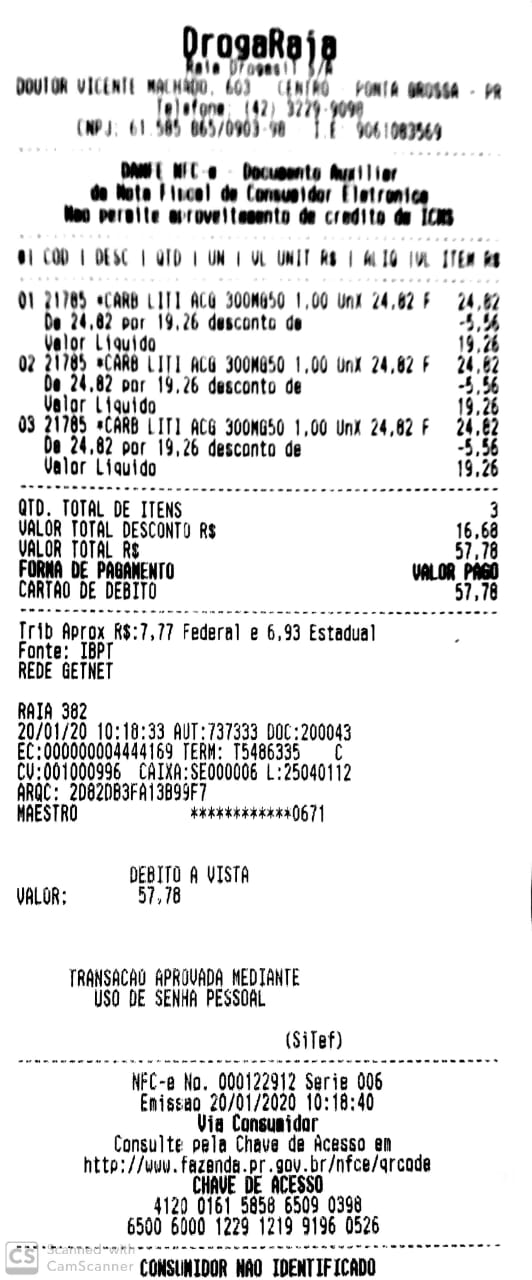This image features a somewhat fuzzy receipt in Spanish, printed on a white background with black text. The store name "Drogaria" appears at the top in bold lettering. Beneath the store name, there is some standard text providing details about the company and their contact information, followed by a section with bolded, darker text. As you continue down the receipt, the list of three purchased items is visible, each accompanied by highlighted and bolded discounts. The first discount is $5.56, followed by another $5.56, culminating in a total discount of $16.68. The initial price of $57.78 is reduced to reflect these discounts. Notably, the receipt mentions that the transaction was completed using a debit visa card. At the bottom, additional information about the retailer, including a website, is provided.